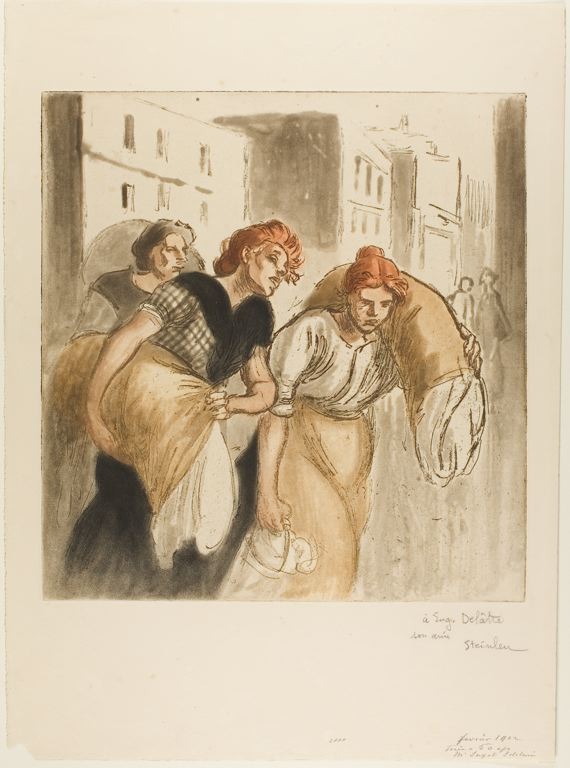The image depicts a vertically aligned rectangular painting or drawing from the early 20th century, featuring three women with distinct appearances and attire. The central area of the artwork is framed within a square outlined in a brownish pencil, set against a white background with faint, possibly indecipherable signatures at the bottom. 

The woman on the left is older, with graying brown hair, dressed in gray clothing. In front of her, towards the center, stands a younger woman with short, styled reddish hair, seemingly moving briskly while carrying a large brown sack with white linen protruding from it. She wears a white top paired with a brown skirt that possibly goes down to her ankles. 

To the right, the third woman has red hair and wears a full-length black dress with a checkered pattern on the right shoulder. She also carries a large sack filled with what appears to be clothing, and in her right hand, she holds a bucket with a handle. 

The background is sketched with outlines of several multi-story buildings, featuring small rectangles that represent windows, with sides shaded in a dark brown hue. This urban atmosphere suggests the women are returning from some chores or errands, possibly carrying personal items or laundry.